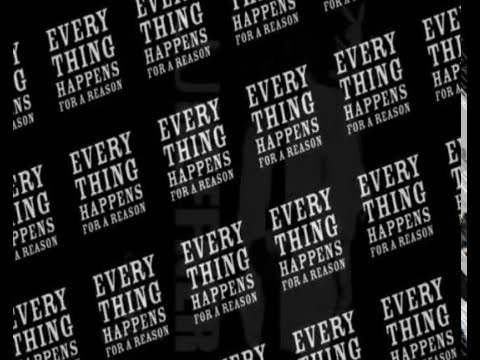The image is a rectangular photograph, slightly wider than it is tall, featuring a repetitive text pattern on a black background. The text reads "everything happens for a reason," arranged in a block where "everything" sits on the top line in bold white font, "happens" below it in a slightly smaller font, and "for a reason" at the bottom in the smallest font. This text block is aligned into a visually cohesive rectangle. 

The pattern repeats diagonally in a grid from the lower left to the upper right, creating four visible rows of this phrase. However, the repetition seems indefinite, fading out at the edges and bottom, giving the impression of continuous repetition. A thin black and white strip borders the right side of the image, disrupting the otherwise consistent pattern. This border is not solid but is distinct enough to be noticeable.

In the background, a hint of another image or perhaps a reflection on a shiny surface is barely discernible. This background contains faint, ambiguous shapes and letters, potentially an F and an R, as well as lighter areas whose exact forms are unclear. Overall, the image conveys a sense of endless repetition and subtle visual complexity against its stark black background.